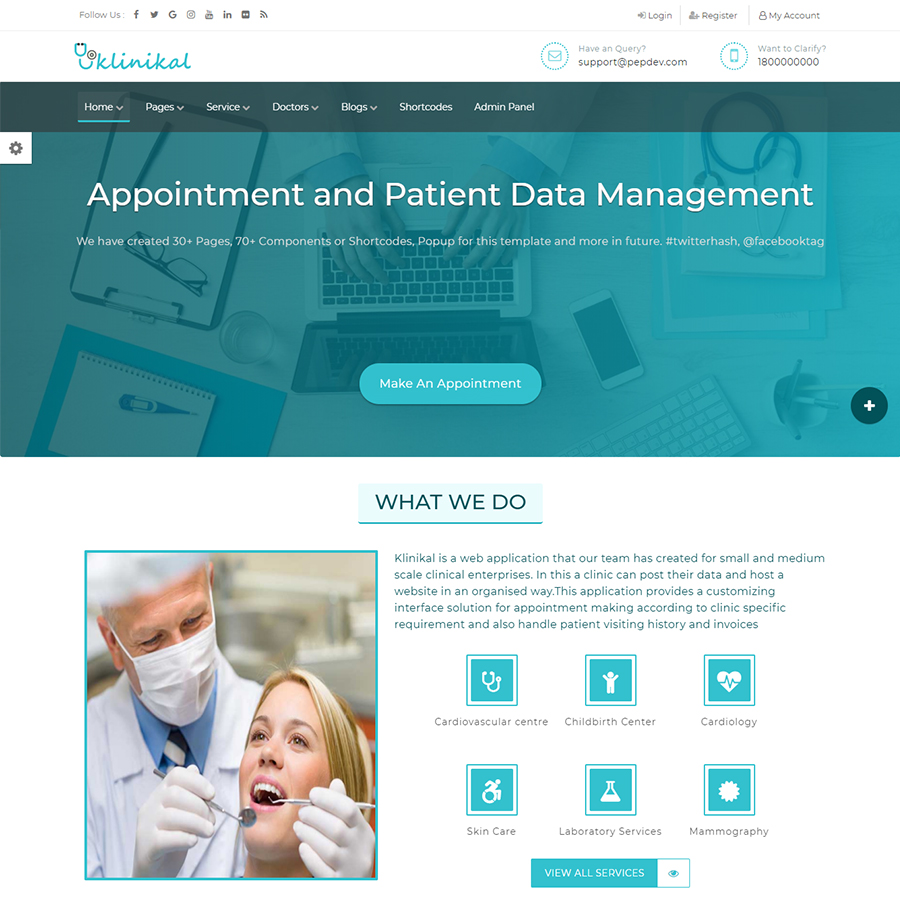This image, likely from a dentist's website, features a comprehensive dashboard themed around appointment and patient data management. The top section includes options to log in, register, and access "My Account." There's also a "Have a Query?" prompt leading to an email contact, complete with a set of phone numbers for further assistance.

The central image displays a professional setting with a person typing on a computer, surrounded by a cell phone, glasses, and a stethoscope, emphasizing a medical or dental environment. The interface prominently showcases a button labeled "Make an Appointment" and highlights detailed text about the appointment and patient data management system.

Additionally, it mentions the creation of over 30 papers, 70+ components or short codes available for this template, with promises of more in the future. The image concludes with six clickable icons at the bottom, presumably for different functionalities or sections of the website, supplemented by hashtags to enhance searchability and user engagement.